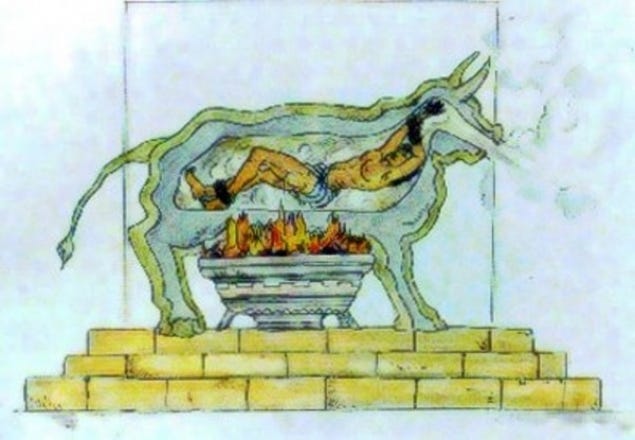The image is a cartoonish drawing depicting a medieval torture device where a person is burning alive inside a bull. This bull, illustrated in a yellowish color with green and blue outlines, is centered in the image, shown in a side profile with the person inside its hollow body. The person is laid out horizontally within the bull, attempting to crawl towards its mouth, with their feet and hands bounded and wearing blue striped bottoms. Below the bull, there is a fire pit with orange and red flames, contributing to the steam coming out of the bull's mouth. The bull stands on three rows of golden yellow bricks. The background behind the scene is a mix of white with lighter bluish shades, featuring some steps at the bottom and a back wall occupying the top part of the image. The overall image has a somewhat blurry, low-resolution appearance.